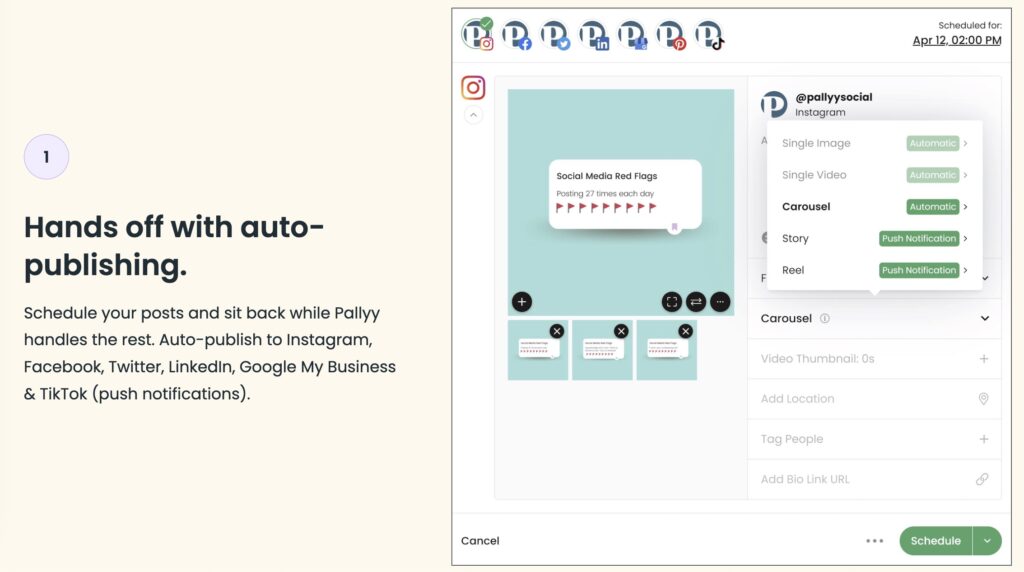**Detailed Caption:**

The image is a screenshot of a publishing website named Pally. The left side of the screen features a cream-colored background displaying a circular icon with the number "1" in light gray. Below this icon is the text "Hands off with auto-publishing," followed by a description: "Schedule your post and sit back while Pally handles the rest. Auto-publish to Instagram, Facebook, Twitter, LinkedIn, Google My Business, and TikTok (push notifications)." This description highlights Pally's seamless auto-publishing capabilities across multiple social media platforms.

In the upper left corner of the image, the Pally logo is prominently displayed. It consists of a capital "P" in white, enclosed within a circle with a green background.

To the right, the image shows a web page interface of the Pally platform. Seven circular icons, each containing a logo, represent various social media platforms: Twitter, Facebook, Instagram, LinkedIn, Pinterest, Discord, and another indistinguishable icon. 

The interface displays a scheduled post example for Instagram, set for April 12th at 2 p.m., illustrating how users can organize their social media content. Additionally, beneath the calendar, there is a layout guide for users, outlining key elements such as avoiding social media red flags and managing posting frequency (e.g., "posting 27 times each day").

Moreover, there is a pop-up menu that offers various post types: single image, single video, carousel, and store reveal, providing diverse content options for auto-publishing. This detailed interface showcases the intuitive and comprehensive functionality of the Pally platform, making social media management effortless for users.